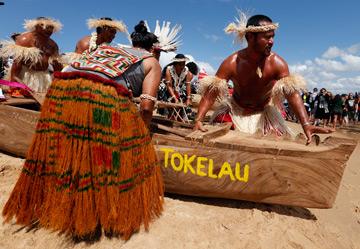The photograph captures a group of darker-skinned individuals, likely Polynesian Islanders or native Hawaiians, on a sandy beach with a clear blue sky above. The central focus is on a wooden boat with "TOKELAU" written in yellow on its side. In the foreground, a woman dressed in a skirt with orange, green, and red hues and wearing traditional bracelets is seen. She appears to be helping three men dressed in white bottoms and adorned with grass headbands and armbands. These individuals, all facing or pointing to the right, seem to be preparing to drag the boat towards the water. There are multiple people in the background, some in similar traditional attire and others in conventional Western clothing, adding to the scene's vivid cultural depiction.